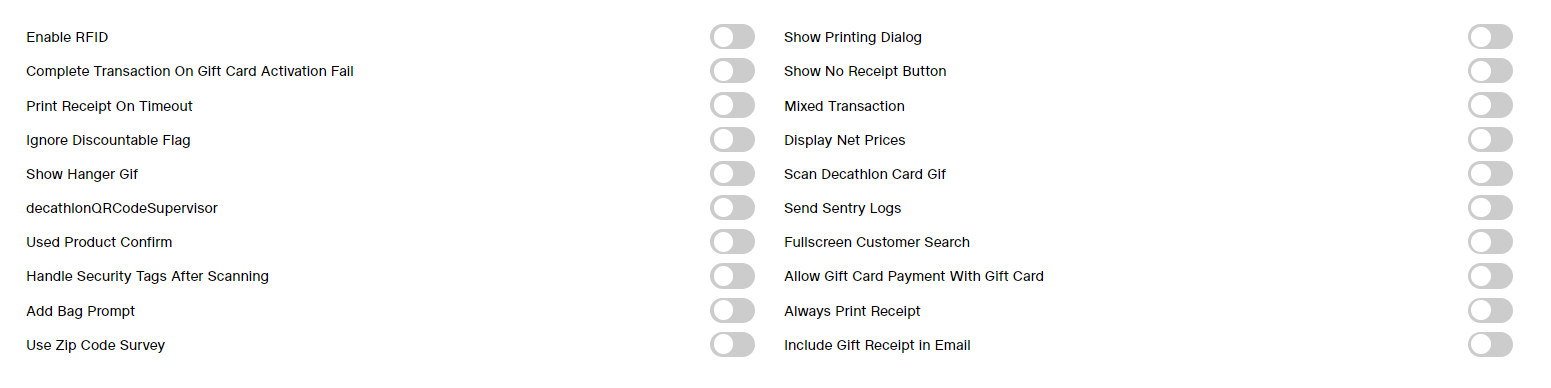The image depicts a settings interface, divided into three distinct columns. Each setting in the interface presents an option with a toggle button next to it, allowing the user to turn the setting on or off. Currently, all the toggles are switched off, as indicated by their gray and white coloring.

In the first column, the settings listed are:
1. **Enable RFID**
2. **Complete transaction on gift card activation fail**
3. **Print receipt on timeout**
4. **Ignore discountable flag**
5. **Show hanger gift**
6. **[Something] with supervisor**
7. **Used product confirm**
8. **Handle security tags after scanning**
9. **Add bag attempt**
10. **Use zip code survey**

The second column contains the settings:
1. **Show printing dialogue**
2. **Show no receipt button**
3. **Miss transaction**
4. **Display net prices**
5. **Scan [something] card gift**
6. **Send security logs**
7. **Full screen customer search**
8. **Allow gift card payment with gift card**
9. **Always print receipt**
10. **Include gift card in email**

Each setting is accompanied by a toggle button for activation, with buttons turned off in this current view. The overall text is in a black font, which contrasts against the white toggles and gray background elements.